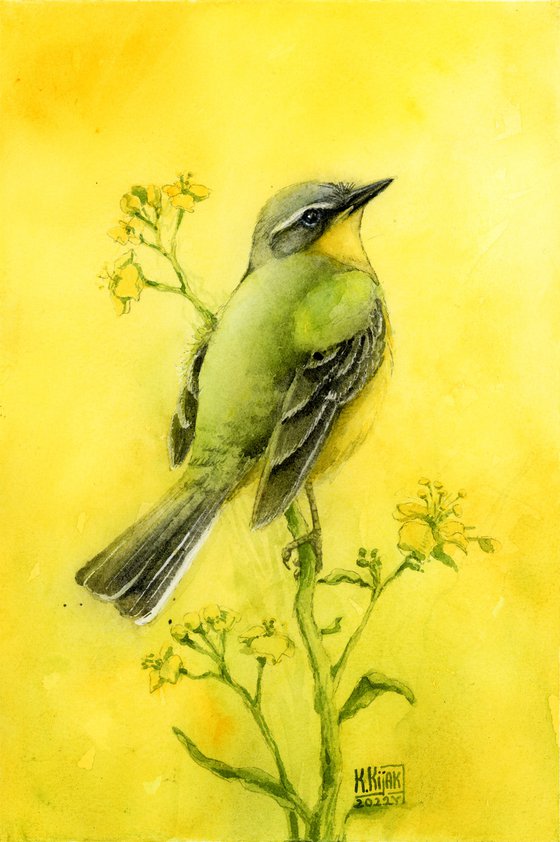This is a vertically oriented, multicolored artistic piece rendered with a vintage aesthetic reminiscent of old illustrations. The background is a mottled array of yellow hues, varying from light lemon yellow to dark orange, with hints of green scattered throughout. Central to the piece is a detailed depiction of a small bird perched on a green branch adorned with leaves and golden yellow flowers.

The bird, facing towards the upper right, features a lime green body and a yellow belly, with a grayish head. Its distinctive features include a black beak and black and white markings around the eyes. The wings and tail feathers are primarily black, with the tail feathers also containing some white. Below the bird, at the very bottom center of the image, is the artist's signature, reading "K. Kijak 2022," indicating the modern creation date despite its antique appearance.